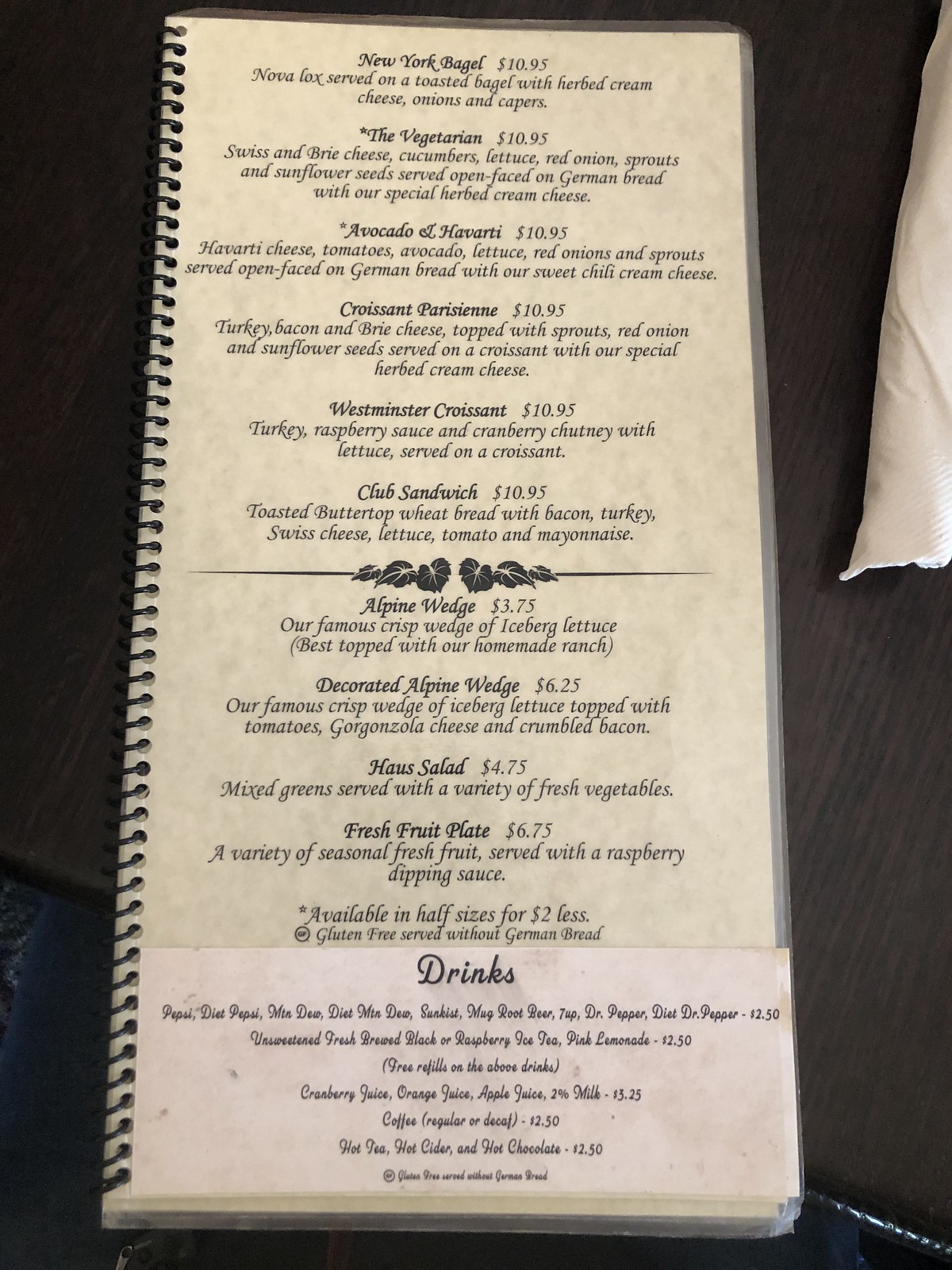On a sleek black table with subtle grain details, a large, vintage-style menu takes center stage. The menu, designed to mimic aged tan parchment, is encased in a spiral notebook with the binding on the left. At the bottom, a slightly brighter white section draws attention to the drinks, still harmonizing with the overall vintage aesthetic. 

From top to bottom, the menu first showcases an array of breakfast options, including a New York bagel, vegetarian avocado and Havarti croissant, Parisienne, Westminster croissant, and a club sandwich, each detailed with their specific ingredients. A single line across the menu and six small leaves mark the transition from sandwiches to salads.

The salad offerings feature an alpine wedge, decorated alpine wedge, house salad, and fresh fruit plate, with half-size portions available for a dollar less and gluten-free options served without German bread. 

The drinks section lists various sodas and unsweetened teas with free refills, along with juices such as cranberry and orange juice, plus an assortment of coffees, hot teas, ciders, and hot chocolate.